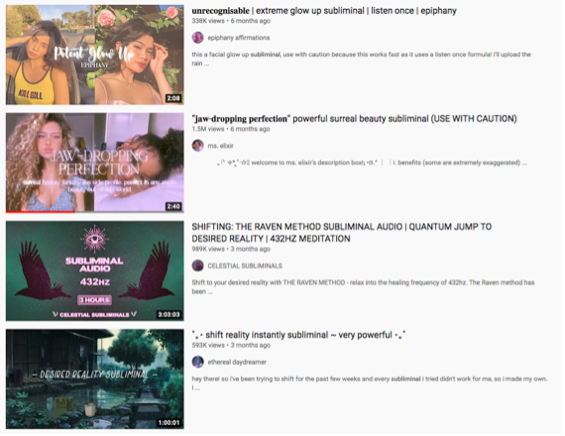This image is a screenshot from a video-sharing website, showcasing four different videos prominently featured on the screen. Along the left side of the image, there are thumbnail previews of each video. On the right side, there are detailed descriptions for each video, which include the title, view count, upload date, the username of the uploader, and a brief synopsis.

The first video, titled **"Unrecognizable, Extreme Glow Up, Subliminal, Listen Once, Epiphany,"** features an image of two sophisticated women standing in front of a floral background. The video is described as offering relaxation through subliminal music.

The second video is named **"Jaw-Dropping Perfection, Powerful Surreal Beauty, Subliminal"** with a cautionary note encouraging careful use. 

The third video, **"Shifting the Raven Method, Subliminal Audio, Quantum Jump to Desired Reality, Meditation,"** features meditation music aimed at relaxation and mindfulness.

The final video is titled **"Shift Reality Instantly, Subliminal, Very Powerful,"** with a runtime of one hour, showcasing another powerful relaxation tool. 

These videos focus on uplifting and relaxing music meant for meditation, with longer-duration options available, such as the third video, which lasts for three hours.